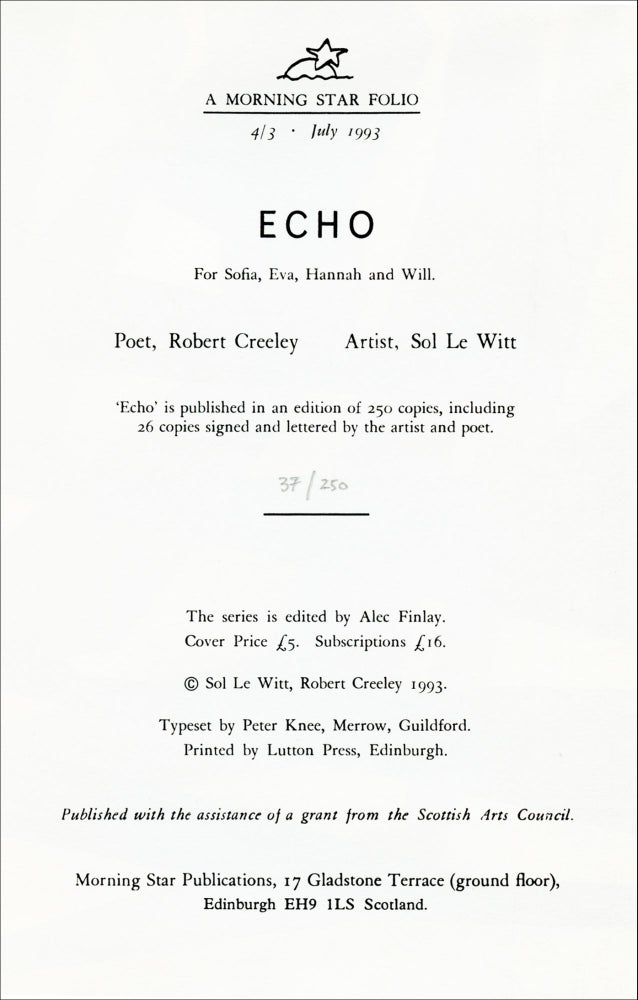This image is a scan of a page or poster that prominently features the word "Echo" in large text. Below it, in smaller black text on a white background, it dedicates the work "for Sophia, Eva, Hannah, and Will." At the top of the document, there's an image of half a sun over water with a star, labeled "A Morning Star Folio," dated "4-3, July 1993." The page continues to detail that the poet is Robert Creeley and the artist is Sol LeWitt. It notes that "Echo" is published as an edition of 250 copies, with 26 of those signed and lettered by the artist and poet, and the specific copy in the image is marked as 37/250 in pencil. The series is edited by Alec Finlay, with typesetting attributed to Peter Key, Anne Merrill, and Guilden. Additional information includes the cover price of £5 and a subscription price of £16. The document was published with assistance from the Scottish Arts Council by Morning Star Publications, located at 17 Gladstone Terrace, Ground Floor, Edinburgh, EH9 1LS, Scotland.